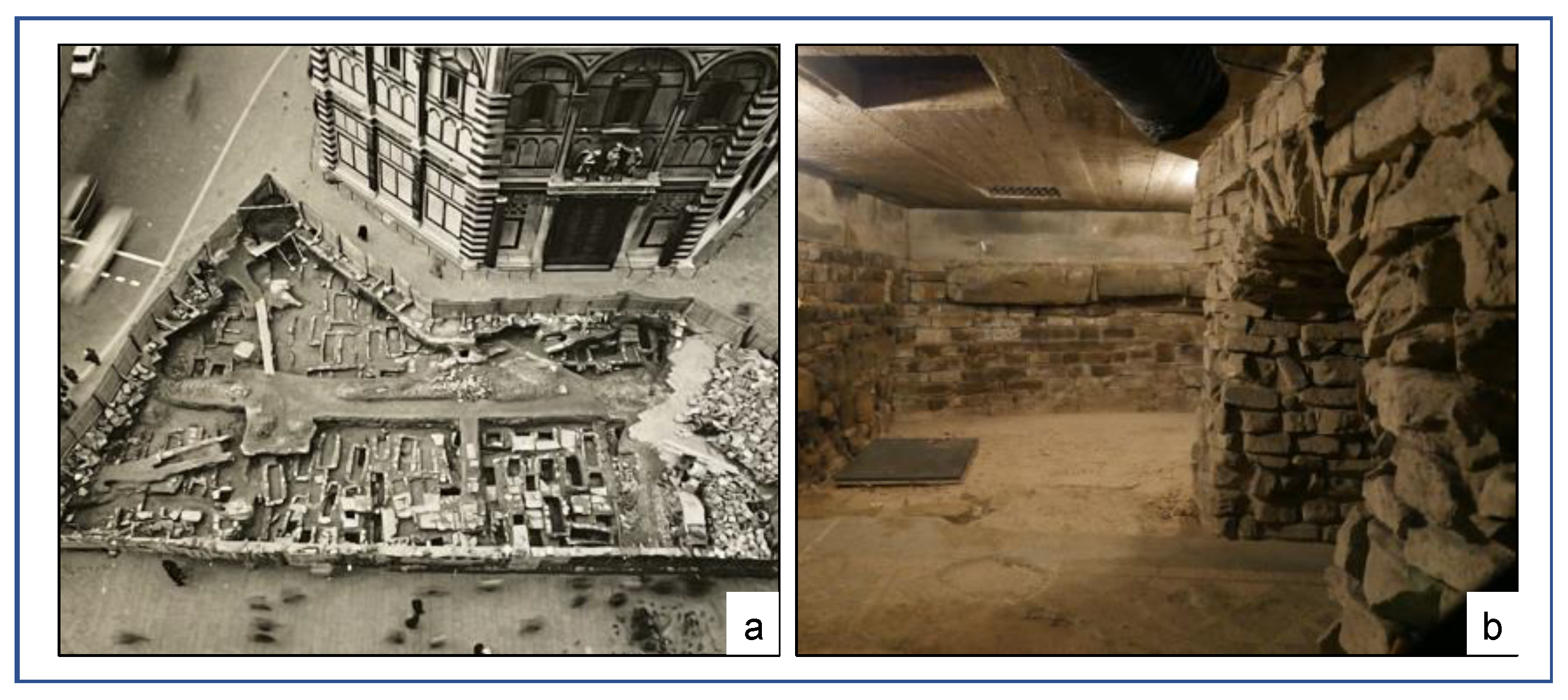The rectangular image features two distinct photographs, each with a different perspective and color tone, bordered thinly in blue on a white background. The left photograph, labeled 'A' in its lower right corner within a white square, is in black and white and offers a top-down view taken from a significant height. This image shows a blurry scene with people walking, a fenced-in area whose contents are unclear, and a large multi-story building positioned at the upper right. The right photograph, labeled 'B' in its lower right corner, captures an indoor, dimly lit scene with a yellowish glow. This photo shows a man-made underground structure with stone walls, archways, and pathways that give it a somewhat eerie appearance. Both photographs together depict contrasting environments – one an external aerial view, the other an interior underground setting.